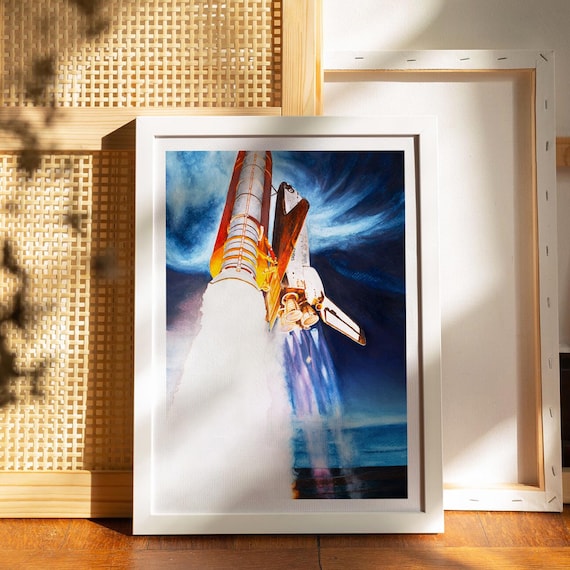A detailed indoor photo captures an art studio bathed in sunlight streaming through a window, casting the shadow of a tree onto a wicker surface behind the main focal point: a vibrantly painted rocket launch. The rocket, primarily white with a vivid red underside, is depicted in mid-launch, still attached to its gear, with a fiery stream of smoke billowing below it and a dynamic blue sky overhead. The painting is set on a white canvas and encased in a white frame, positioned prominently against a white wall with matching trim. To the right of the rocket painting, a blank canvas turned away from the camera shows the back with visible staples. The room features light honey-colored wooden floors. In the background, there's a wooden divider wall with see-through holes, accompanied by a plant on the left-hand side, adding to the serene but creative ambiance.